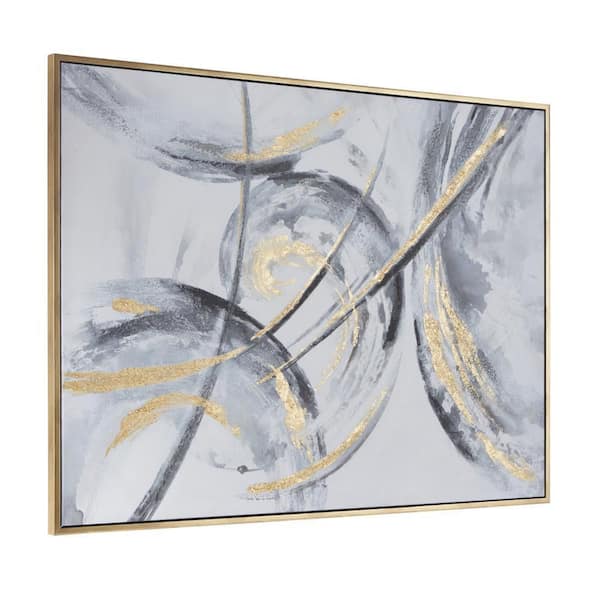The image depicts an abstract painting encased in a thin, brass-colored frame, set against a solid white background. The painting features a light gray backdrop adorned with dynamic swirls and strokes in shades of black, dark gray, and gold. The composition appears highly abstract, with swirling patterns suggesting fragmented circles or comma-like shapes, and several thin, curving lines extending from the top right towards the bottom left, covering about 75% of the canvas. Blank spaces in the top left and bottom center reveal more of the gray background. The frame and painting are slightly tilted, with the left side closer to the viewer, enhancing the sense of depth and movement within the artwork. Thin black lines and golden flakes add intricate details, contributing to the overall abstract and contemporary feel, making it a piece worthy of an art gallery or museum.